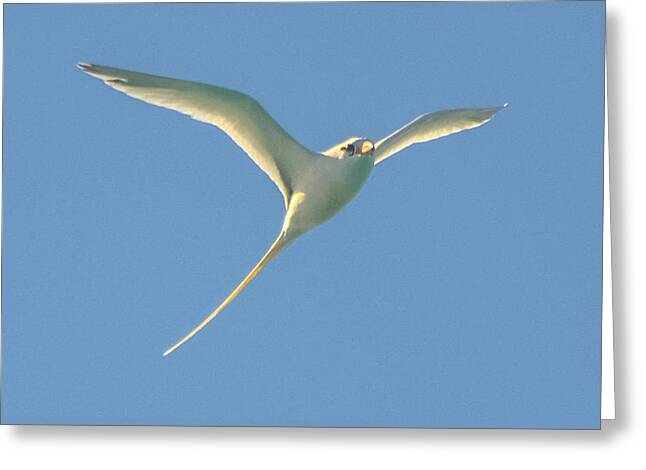This image features a detailed portrayal of a bird soaring through a clear, light blue sky. The background is completely devoid of clouds, emphasizing the undisturbed aerial scene. The bird is centrally positioned and depicted in mid-flight with its wings fully spread. The distinctive wingspan is impressive, and the bird's posture suggests it is intent and determined, possibly having spotted a distant target.

The bird’s body is predominantly white, with gray shades under its wings and belly. It possesses a long, thin white tail that adds to its elegant flight profile. Notably, one can see the right side of the bird, including its black eye and short, thick, orangish-yellow beak. This side view captures the bird angling slightly upward to the right, with its tail pointing downwards to the left. The overall effect is one of serene motion and determined grace against a solid, bright blue sky. The representation, whether a painting or a digitally created image, uses a palette of blue, white, gray, and accents of orange and yellow to bring the bird to life against its sky-blue background.